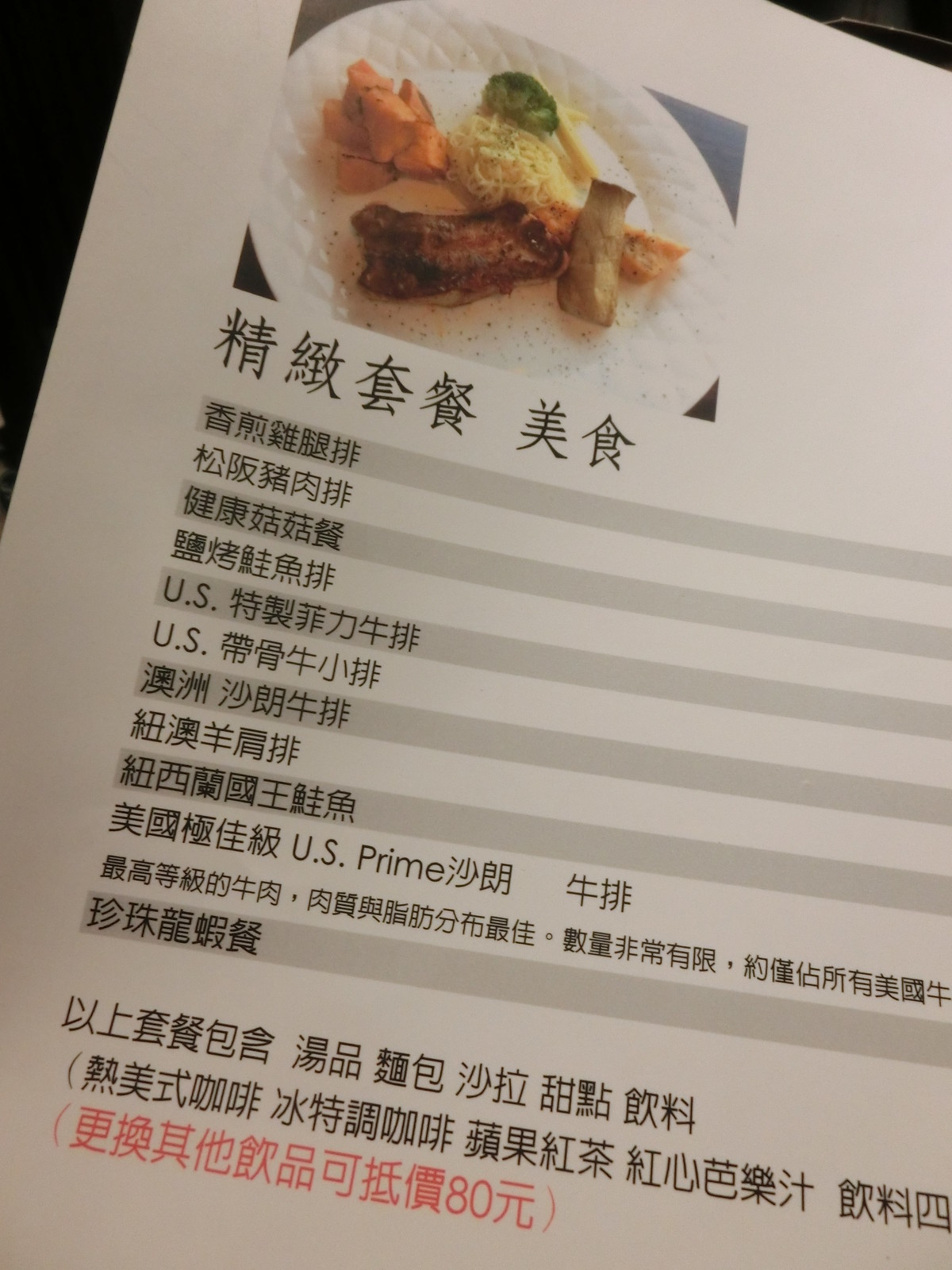The image depicts a Chinese food menu set against a black background. Centered on the black backdrop is a white piece of paper. At the top of this paper is a rectangular section featuring a vivid photograph of various Asian dishes including noodles, broccoli, and possibly carrots, with an assortment of meat positioned prominently in the foreground. 

Below the image, there are twelve lines of text written in Chinese characters. Notably, the fifth, sixth, and eighth lines include the term "U.S." in English, with specific mentions such as "U.S. prime." Beneath these lines, there are three additional lines of Chinese text. The final line is distinct, written in bright red font and enclosed in parentheses, contrasting with the black font used in the rest of the text.